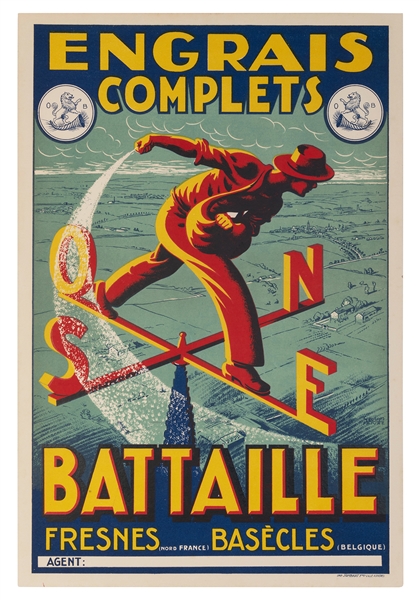This historical French advertisement poster for fertilizer depicts a vivid scene featuring a farmer spreading fertilizer by hand from a satchel. The farmer, illustrated in striking shades of red and yellow, stands atop a weather vane, symbolizing the comprehensive fertilization of his entire farm in every direction—North, South, East, and West. The letters on the weather vane use a French-style typology, with "O" representing West. The text, rendered in gold writing, highlights the product as "Engrais Complète" (Complete Fertilizer), indicating its all-encompassing nature. Additional details include a medallion of a lion rearing up on a cornucopia, flanked by the letters "OB", and the backdrop consists of a serene pale grayish blue landscape. Names and locations such as Bataille, Fresnes, Noro, France, and Bassaclès, Belgique are noted, suggesting regions of distribution or production. This meticulously designed poster not only promotes the product's efficacy in aiding growth under any conditions but also stands as an artistic and cultural artifact with its rich color palette and intricate details.